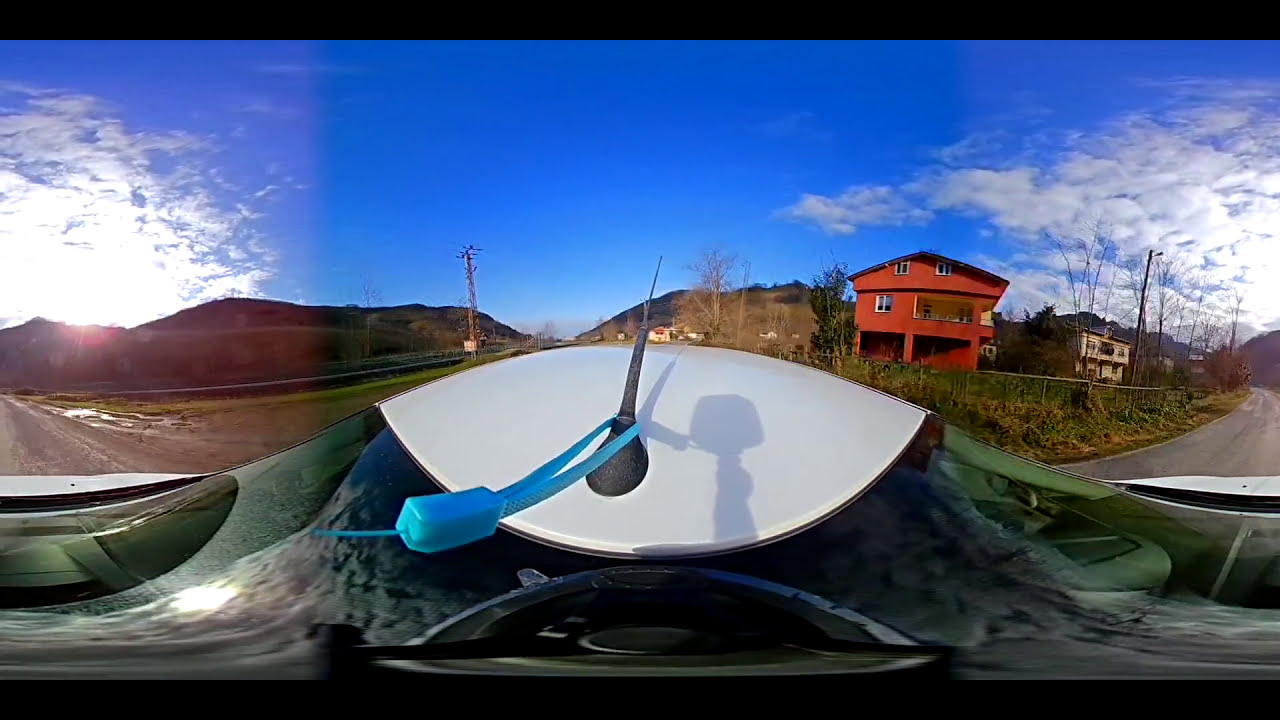This vibrant outdoor image, taken from the perspective of a drone hovering over a roadway, captures a diverse and colorful landscape bathed in the light of mid-day. The sky, painted a vivid blue, is sprinkled with white, wispy clouds and stretches across the top of the image. The foreground prominently features the front end of a black and green drone, with a blue rectangular device extending from an antenna towards the left. The drone reflects the sky, giving a shiny appearance with flecks of green and black.

Central to the image is a red, three-story farmhouse surrounded by lush, green grass and high weeds. A brown house stands adjacent to the red one, both structures nestled against a backdrop of rolling hills and mountains. Intersecting the frame is a road that runs along the left side, where a crane or lamppost rises into the sky. Towards the center, there is a metal fence, adding another layer of detail to the pastoral setting.

Overall, the composition paints a detailed and vibrant scene of rural architecture and natural beauty, captured from a unique aerial viewpoint.